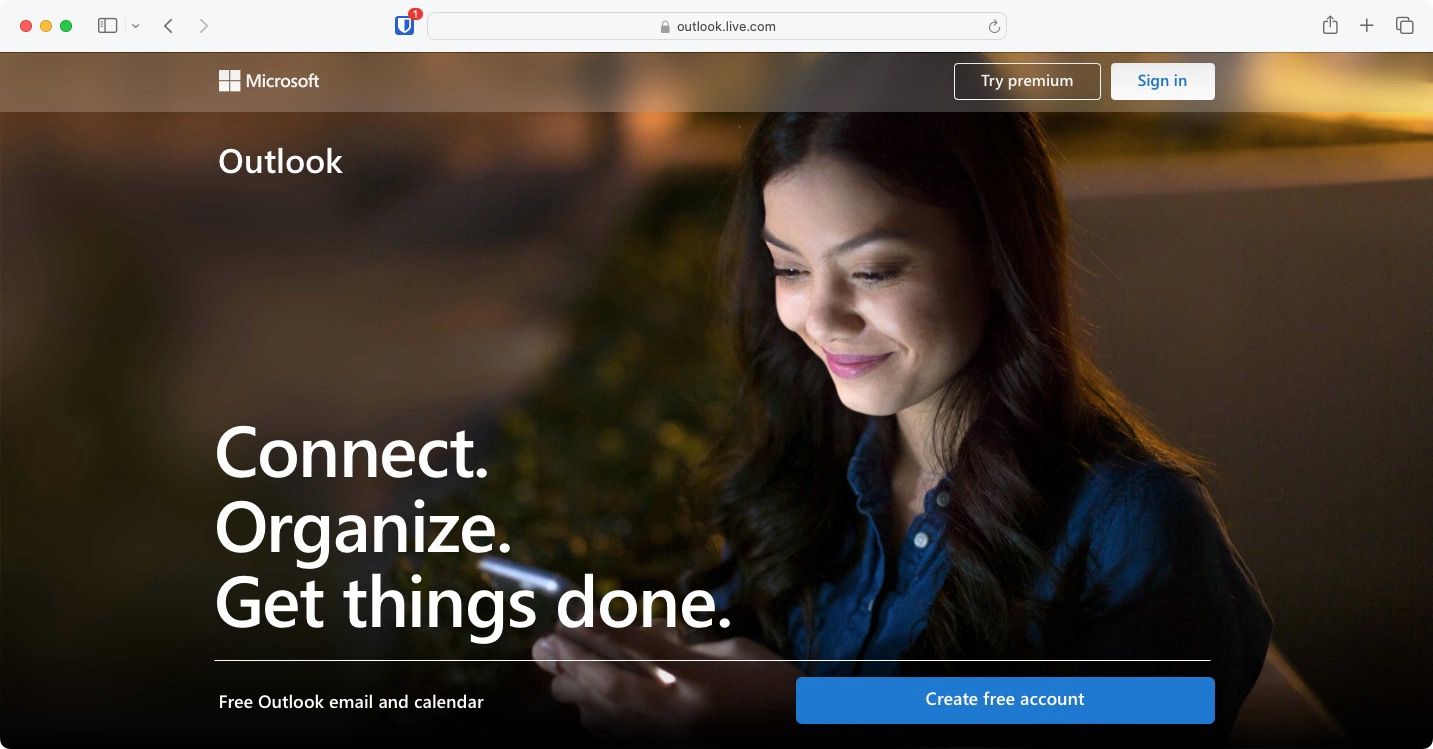A screenshot of a macOS desktop window displaying the homepage of Microsoft Outlook (outlook.live.com) is open in the Safari browser. In the address bar, the URL is clearly visible, confirming the site being visited. Dominating the webpage is a stock image of a woman in a dimly lit, open-space office environment, engrossed in her phone. The light from her phone subtly illuminates her face, providing a focal point in the otherwise shadowy setting. Across the image, bold text reads, "Connect, organize, get things done," promoting Outlook's email and calendar services. Below this tagline, a prominent blue button invites users to "Create free account," alongside another statement offering free email and calendar options. At the top of the page, two additional buttons, "Try premium" and "Sign in," facilitate easy navigation for returning users or those seeking upgraded features. The Safari browser interface shows elements such as tabs and sharing options, contributing to a comprehensive snapshot of the browsing experience. Notably, such atmospheric stock photos with low lighting are an atypical but engaging choice for web interfaces.